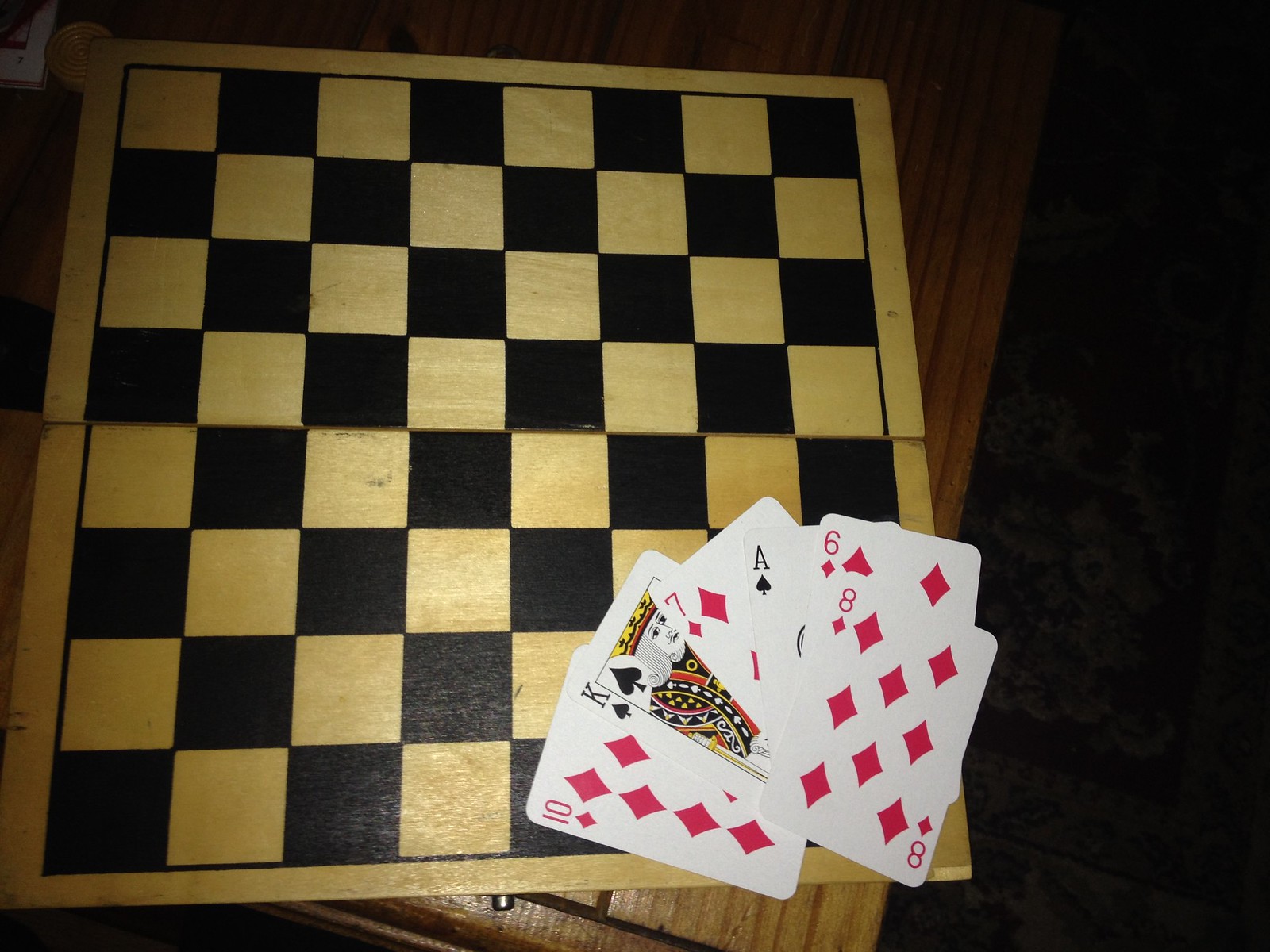The image depicts a wooden, folding checkerboard (or chessboard) resting on a wooden table. The checkerboard consists of alternately placed black and white squares. Positioned in the lower right corner of the checkerboard is a fanned-out hand of six playing cards. The cards, starting from left to right, are as follows: 10 of Diamonds, King of Spades, 7 of Diamonds, Ace of Spades, 6 of Diamonds, and 8 of Diamonds. Despite the presence of high-value cards like the Ace, the hand lacks any meaningful combination such as pairs or straights. The scene appears to be illuminated by a camera flash, creating a stark contrast between the brightly lit checkerboard and cards, and the darker background.